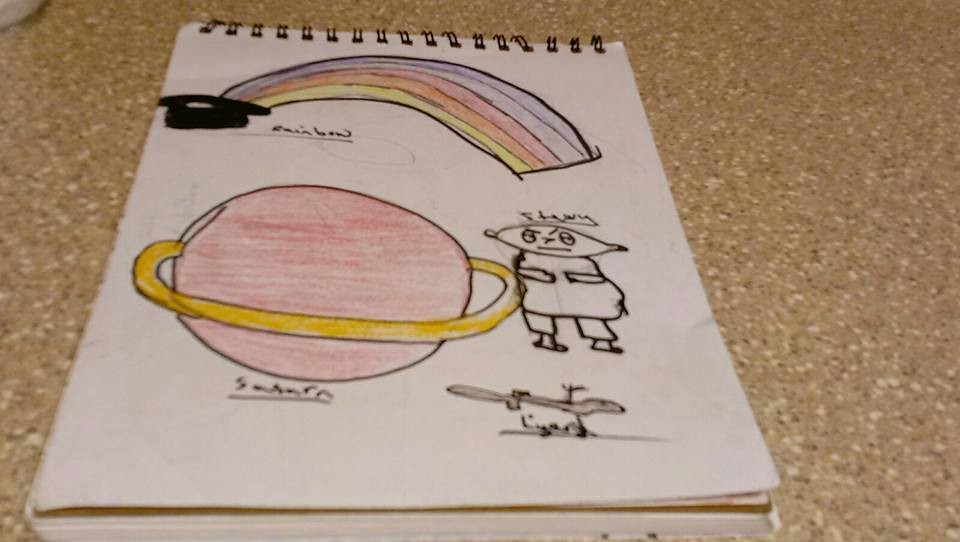A vibrant sketch adorns the white page of a ring-bound sketching pad, set against a backdrop of beige carpet. Captivatingly childlike artistry depicts a colorful scene. At the top of the page, a rainbow arching from a simple black pot of gold spans the composition in hues of violet, orange, and yellow, defying the conventional ROYGBIV spectrum. To the left and slightly below this, the pot of gold nestles snugly. Dominating the central area is a playful rendition of Saturn, its rings meticulously detailed. Next to the planet, a uniquely characterized figure stands out—a cartoon character with a football-shaped head, a round potato-shaped body, thin arms and legs, and a striking bald appearance. Above this whimsical figure, the name "Stewie" is inscribed, revealing the character's identity. Beneath him, a slender, long-tailed lizard adds an additional layer of charm to the drawing.